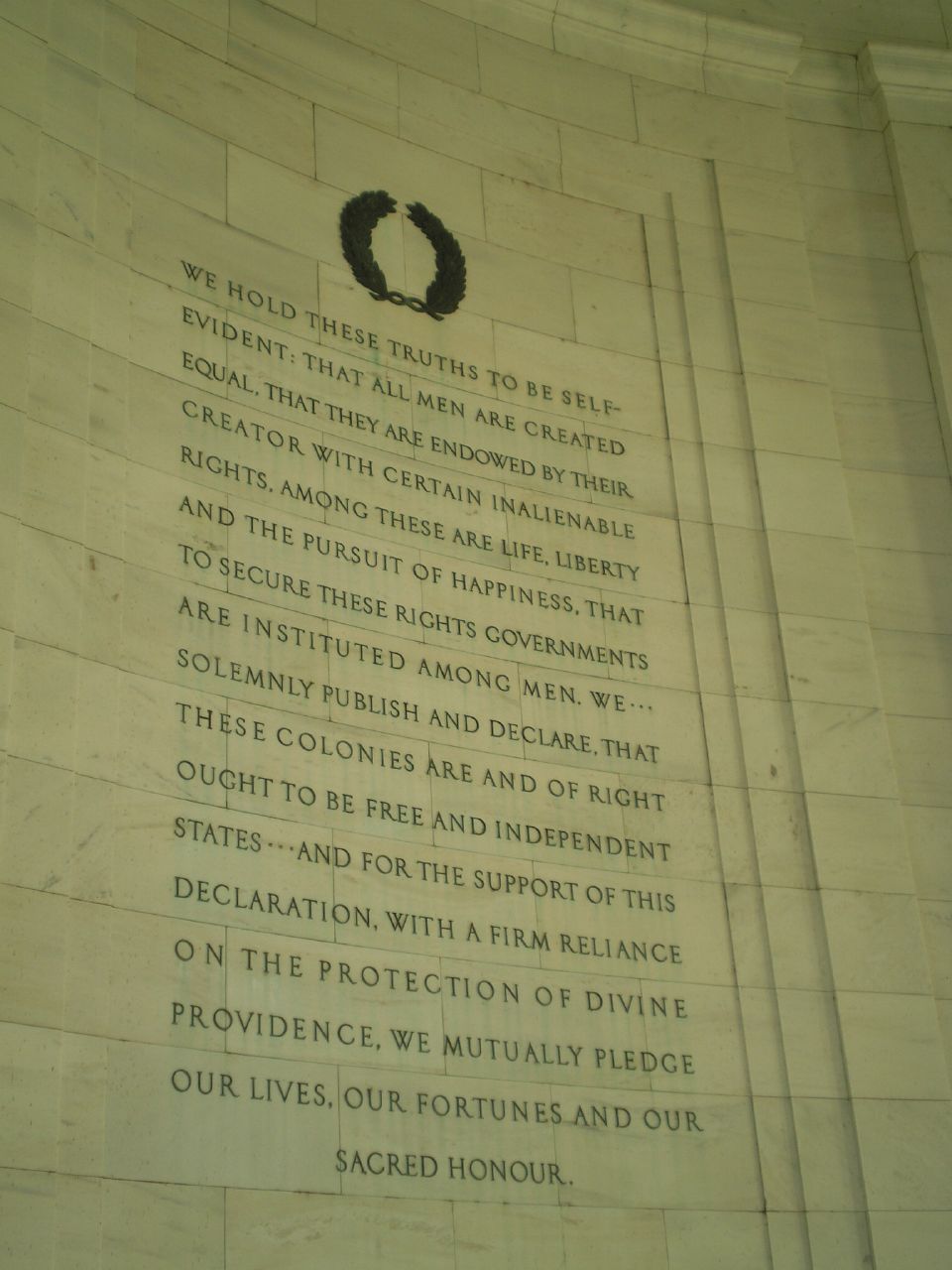The photograph captures a close-up of a curved wall inside a stone building, potentially a rotunda or a museum. The wall appears to be made of grayish-white marble or granite, giving it a dignified and monumental look. At the top of the wall, there is a stylized metal symbol resembling two holly branches or feathers tied together with a chain, presented in black. Below this symbol, a significant engraving runs from the top to the bottom of the wall. The text, carved in a bold, all-caps font, begins with the iconic words, "We hold these truths to be self-evident, that all men are created equal," from the Declaration of Independence. The inscription continues, outlining essential principles of liberty and the purpose of government, ending with the profound commitment: "We mutually pledge our lives, our fortunes, and our sacred honor." Additionally, a pediment is visible at the top of the image, along with part of a column on the upper right side of the wall, adding to the architectural grandeur of the setting.